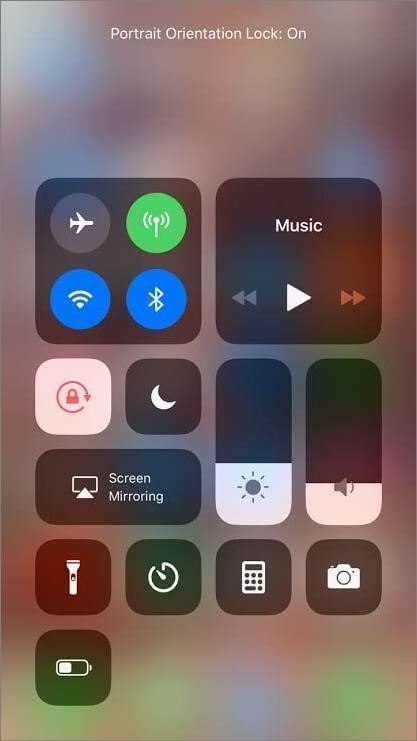The image displayed on the cell phone screen captures a user’s control center with the portrait orientation lock feature activated, as indicated by the "Portrait Orientation Lock: On" message at the top. The background is slightly blurred, highlighting the active control center pop-up.

At the top left corner of the control center, there's a square icon containing four circles, each representing different modes: airplane mode, signal strength, connectivity, and screen rotation lock, displayed in that order. Directly below, there is a set of music control buttons, including play, fast forward, and rewind options.

To the right, there’s a section with additional utilities. This includes a lock icon for securing the screen and a return icon. Below these, a square with a moon symbol represents the Do Not Disturb mode. Next to it, a rectangle labeled "Screen Mirroring" indicates the option to mirror the phone's display to another device.

The control center also has sliders for adjusting brightness and volume. The brightness slider allows the user to lighten or darken the screen, while the volume slider enables adjusting sound levels.

In the bottom row, a series of quick access icons are visible: a flashlight icon for activating or deactivating the flashlight, a timer icon for setting a countdown, a calculator icon for quick calculations, and a camera icon for easy access to the camera. At the very bottom, a battery icon displays the current battery level, shown to be half full.